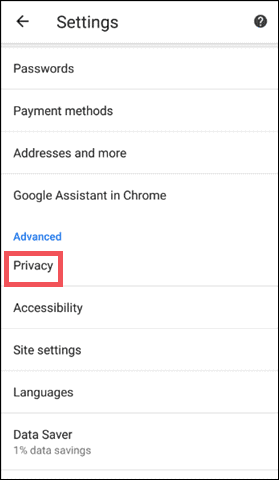This detailed caption describes an image captured in portrait mode with a thin black border surrounding it. The focus of the image is a highlighted section within the settings of a particular application, likely a web browser. 

At the top left corner of the screenshot, there is a back arrow icon. Adjacent to it, in bold black text, is the word "Settings." On the top right corner, there is a circle with a question mark inside, presumably for help or additional information.

Below the header, a gray line separates the title from the main settings menu, which consists of several rows:

1. **Passwords**
2. **Payment Methods**
3. **Addresses and More**
4. **Google Assistant in Chrome**

Each row is divided by thin gray lines. The screenshot specifically emphasizes the "Google Assistant in Chrome" row, indicating this is where the user's current focus lies. 

Beneath this, in blue, is the word "Advanced," suggesting a clickable link for more options.

Another gray line leads to the next section titled “Privacy,” which the user has marked with a red rectangle, marking it as particularly significant in the context.

Subsequent rows include:
- **Accessibility**
- **Site Settings**
- **Languages**

In the bottom left-hand corner of the screenshot, there is a "Data Saver" option indicating “1% data savings.” 

Overall, this image captures the settings interface, with a specific emphasis on the privacy settings, highlighted by the red rectangle added by the user. This meticulous layout visually guides the viewer through the settings menu, indicating the prioritized sections.